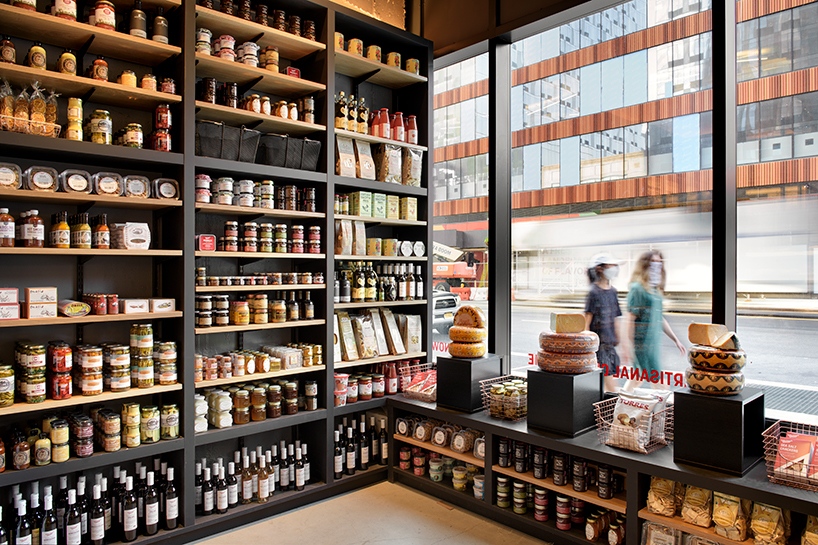The image depicts the interior of an old-world style specialty shop with meticulously decorated black shelves brimming with an array of products. On the left side, shelves are densely stocked with various items including glass bottles, jars, cans, paper boxes, and designer boxes potentially containing cakes, bakery items, drinks, sauces, condiments, and even pasta like macaroni. To the right, a large stained glass window with copper strips and individual clear panes overlooks a busy street. Below this window are two black pedestals displaying bowls and two additional shelves housing more goods. The scene outside the window is bathed in daylight, revealing vehicles on the road and buildings with large glass windows. Two women, one in a blue dress and the other in a green dress, both wearing face masks, walk by, slightly blurred. There is also some writing on the window, possibly the store’s name, adding to the quaint and charming atmosphere of the shop.